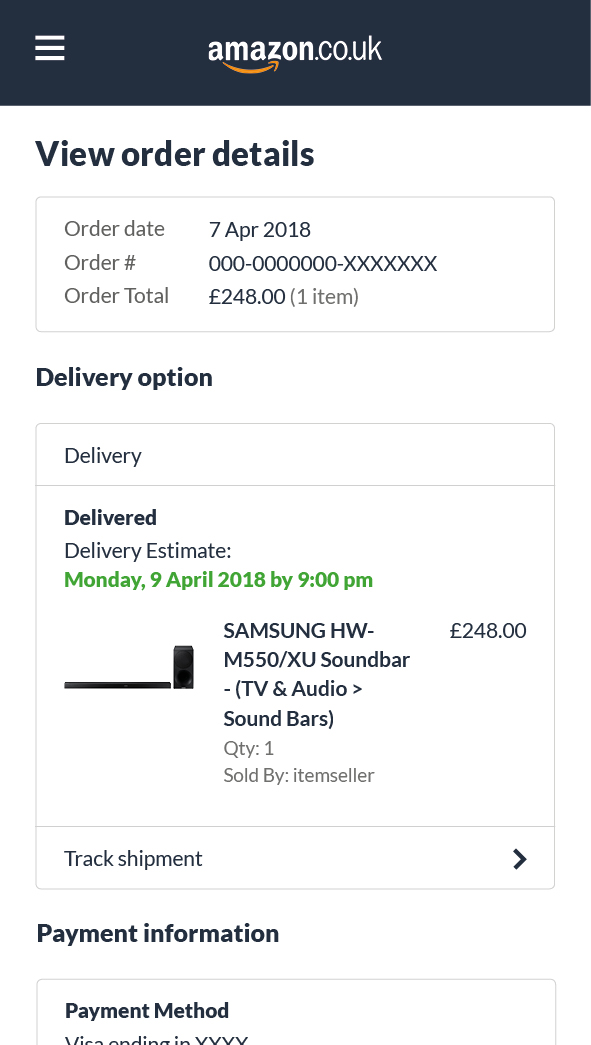The image is a rectangular screenshot with its long side extending from top to bottom, displaying an Amazon order summary. At the top, there's a dark gray border featuring a hamburger menu icon on the left and "Amazon.co.uk" in white text centered, with the Amazon logo beneath it.

Directly below, in bold white text, it reads "View Order Details." This is followed by a thin gray line creating a boxed section that provides order specifics: 

- **Order Date:** 7th of April, 2018
- **Order Number:** [specific number]
- **Order Total:** £248
- **Item Quantity:** 1

The background of the image is predominantly white. Below the order details, the section title "Delivery Option" is printed in black. Underneath, another thin gray line frames the delivery specifics:

- **Delivery Estimate:** Monday, 9th April, 2018 by 9 p.m.
- **Product:** Samsung HW-M550-XU Soundbar TV and Audio Soundbars
- **Quantity:** 1
- **Sold by:** [Item Seller]
- **Price:** £248

Following this, there's a section for tracking shipment and additional payment information.